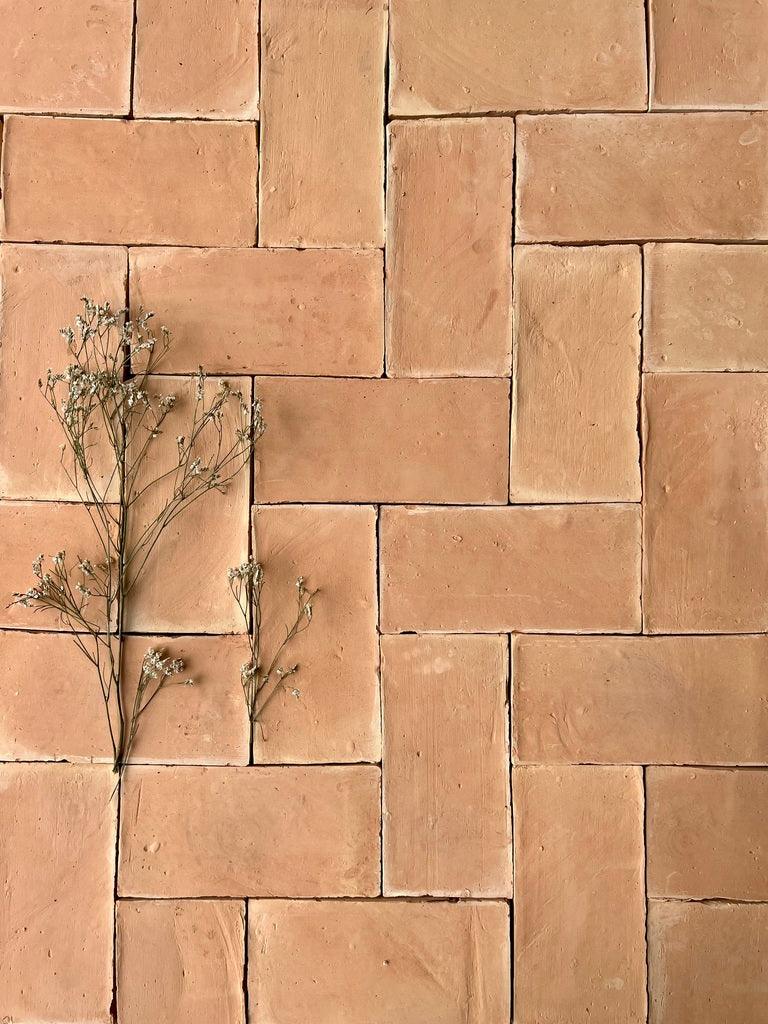This detailed color photograph, set in portrait orientation, captures a brick floor composed of rectangular pavers that resemble patio stone pavers. The bricks, identical in their tan color with white-edged wear showing various chip and pit marks, interweave in a striking zigzag pattern across the entire image. The arrangement includes staggered layouts of vertical and horizontal bricks creating an even, intricate design. The bricks vary slightly in shades of brown, showcasing a natural earthy palette without grout between them. Centrally and towards the left side of the image, two dried stems extend vertically — the larger on the left and the smaller on the right, each adorned with multiple white dried flowers. Their similar appearance indicates they are likely from the same plant species, adding a delicate touch to the rugged texture of the brick floor. The photograph, embodying photographic realism, highlights the contrast between the organic vulnerability of the dried flowers and the sturdy durability of the brick pattern.